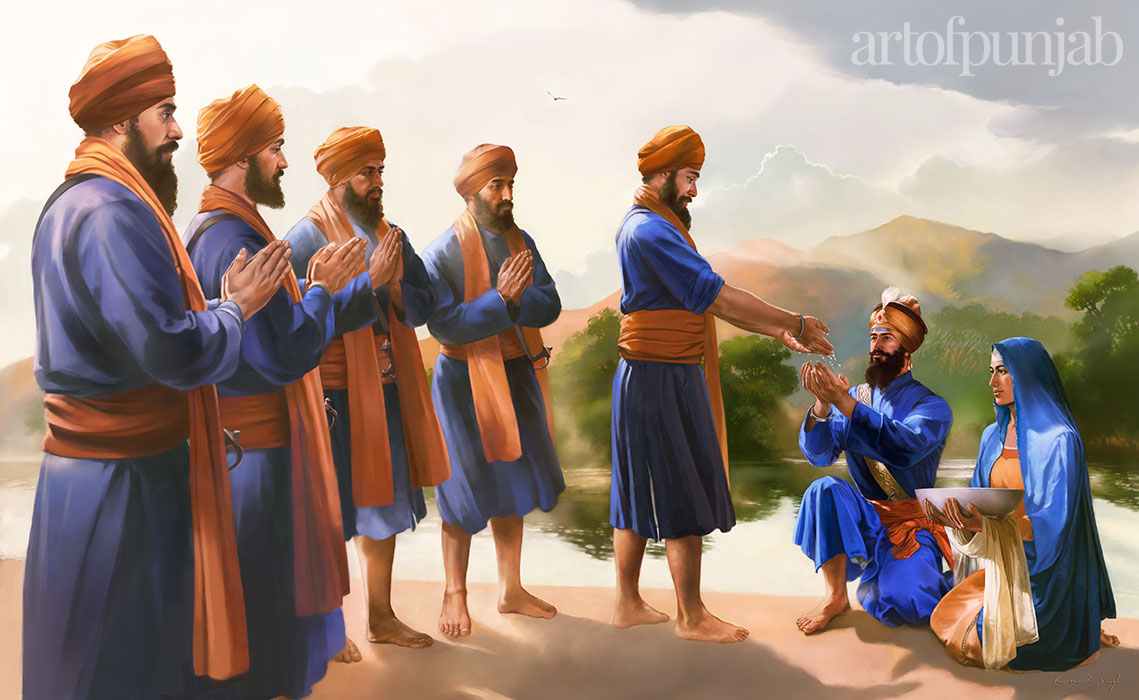This digital artwork, titled "artofpunjab" in lowercase letters located in the upper right corner in light gray, vividly portrays a ceremonial scene with rich cultural elements. The backdrop displays a serene landscape with white and grayish clouds, distant brown mountains, a tree line, and a body of water, enhancing the composition. In the center, a man wearing a blue satin robe and an orange turban adorned with a jewel is kneeling, holding his hands out to receive water. Beside him, a woman dressed in a blue robe and an orange dress, reminiscent of the religious figure Mary, is also kneeling and holding a large ceramic bowl. This central man is flanked by another man, similarly attired in a blue robe, brown head cloth, and brown scarf, who is seen pouring water onto the kneeling man's hands. To the left, a group of six men, each with a black beard and donning blue robes, orange turbans, orange sashes, and brown headgear, stand with their hands together in a prayer position, suggesting a ritualistic or wedding ceremony. The intricate details of the clothing, the ceremonial actions, and the tranquil yet dynamic background all contribute to the storytelling and cultural depth of the image.